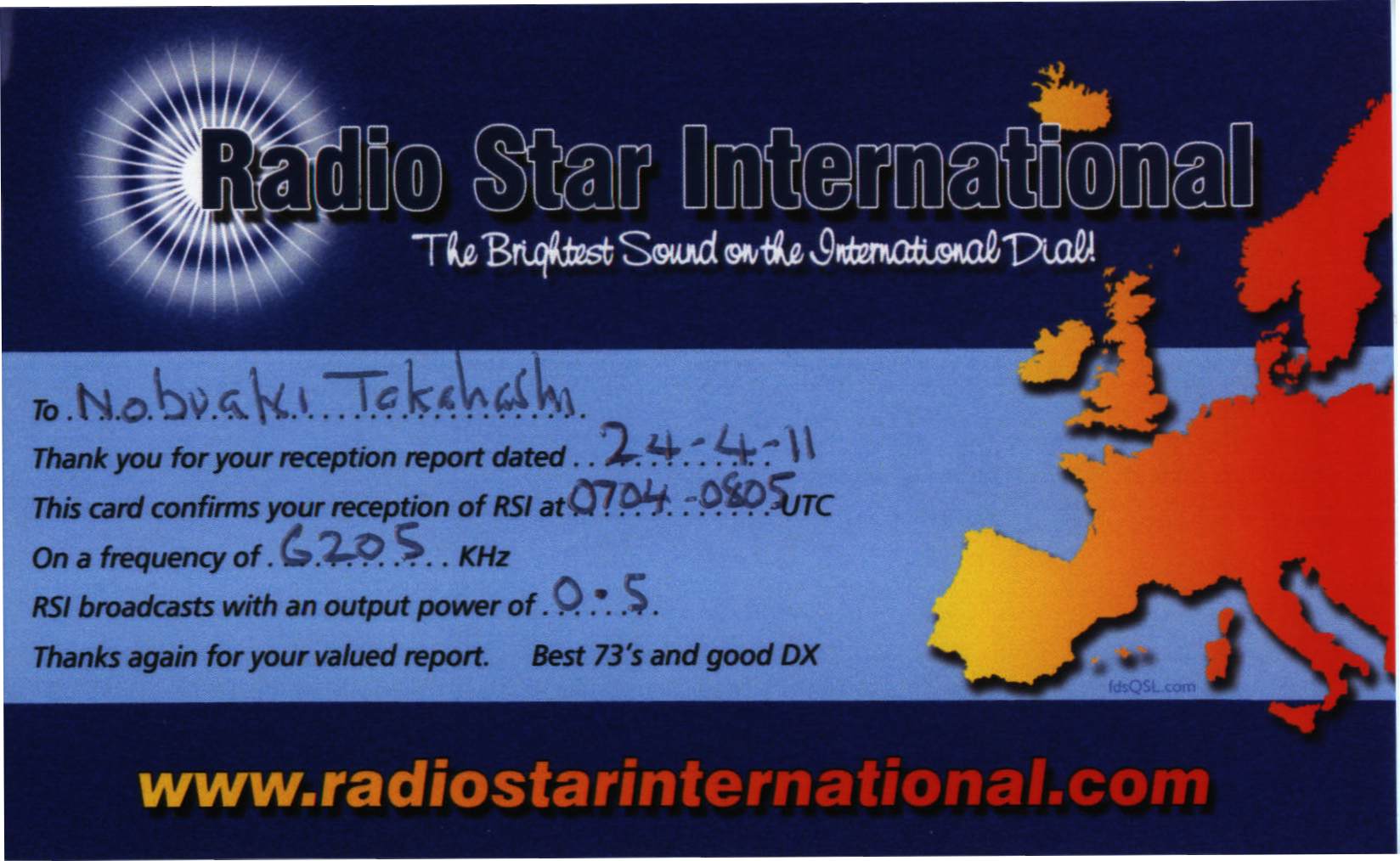Against a backdrop of deep navy blue transitioning to dark purple at the top, this striking poster features a radiant design: white lines emanating from a central dark blue-black circle, encircled by a whitish ring. Prominently displayed at the top in bold black lettering is "Radio Star International," with the tagline "the brightest sound on the international dial" written underneath in elegant white cursive.

To the right, a vivid map of Europe spans from brick red near Scandinavia—depicting countries like England, Ireland, Sweden, Finland, and Italy—to golden yellow towards Spain. The map's vibrant colors fade seamlessly from right to left. Superimposed on this map are handwritten notes, reading: "Nobuaki Toka Shihei, thank you for your reception report dated 24-4-11. This card confirms your reception of RSI at 0704-0805 UTC on a frequency of 6205 kHz. RSI broadcasts with an output power of 0.5 kW. Thanks again for your valued report. Best 73's and good DX."

At the very bottom, amidst a darker blue section, the website "www.radio-star-international.com" is displayed, its color transitioning from gold-yellow to red as it moves from left to right.